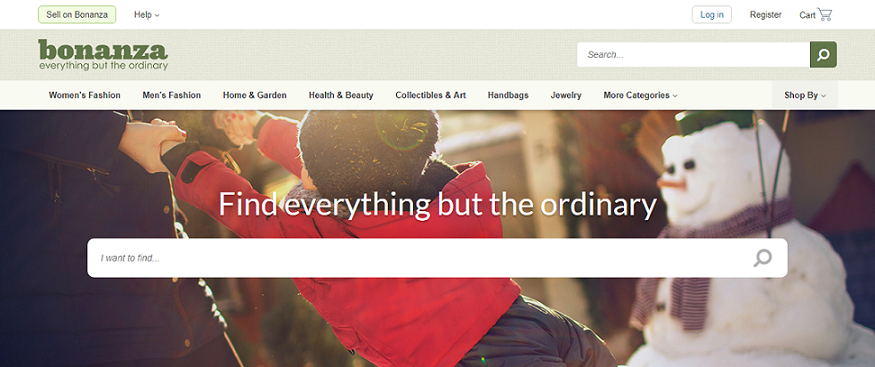This image is a screenshot taken from the Bonanza website, featuring the company's tagline "Everything but the ordinary." At the very top, there are navigational buttons including "Sell on Bonanza," "Help," "Log In," "Register," and a shopping cart icon. Additionally, there's a prominent search bar with a magnifying glass icon, denoted by the word "Search," allowing users to enter their queries.

On the left side, beneath the company name, there is a series of clickable category links like "Women's Fashion," "Men's Fashion," "Home & Garden," "Health & Beauty," "Collectibles & Art," "Handbags," "Jewelry," and a "More Categories" link with a dropdown menu indicated by an arrow. These categories aid users in navigating various sections efficiently.

Further down the page, another dropdown menu is available under the "Shop" section, expanding to show more options when clicked.

The central part of the image features a winter scene: an adult woman, identified by her smaller hands, is depicted playing outside in the snow by swinging a young boy, who is joyfully donning a green cap, a red sweatshirt, blue snow pants, and winter boots. In the background, a cheerful snowman with a carrot nose adds to the festive and playful ambiance of the scene.